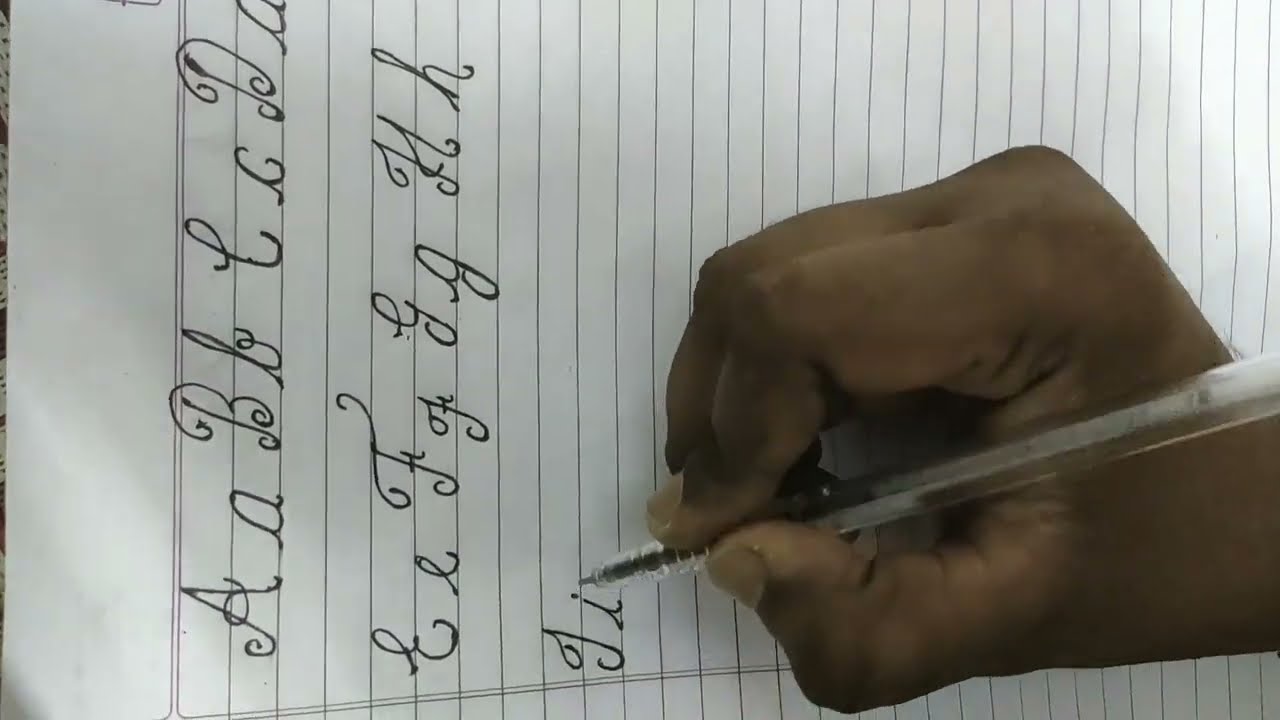The image depicts a close-up of a person's hand, with brown skin, holding a transparent plastic pen with a black tip. The pen is actively writing on a sheet of lined notebook paper. The orientation of the image is sideways, causing the lines on the paper to run vertically. The individual is practicing cursive writing, meticulously forming uppercase and lowercase letters side by side. The sequence of letters written so far spans from A to I, with uppercase letters taking up two lines each. The ink used is black, and the next letter to be written appears to be J.